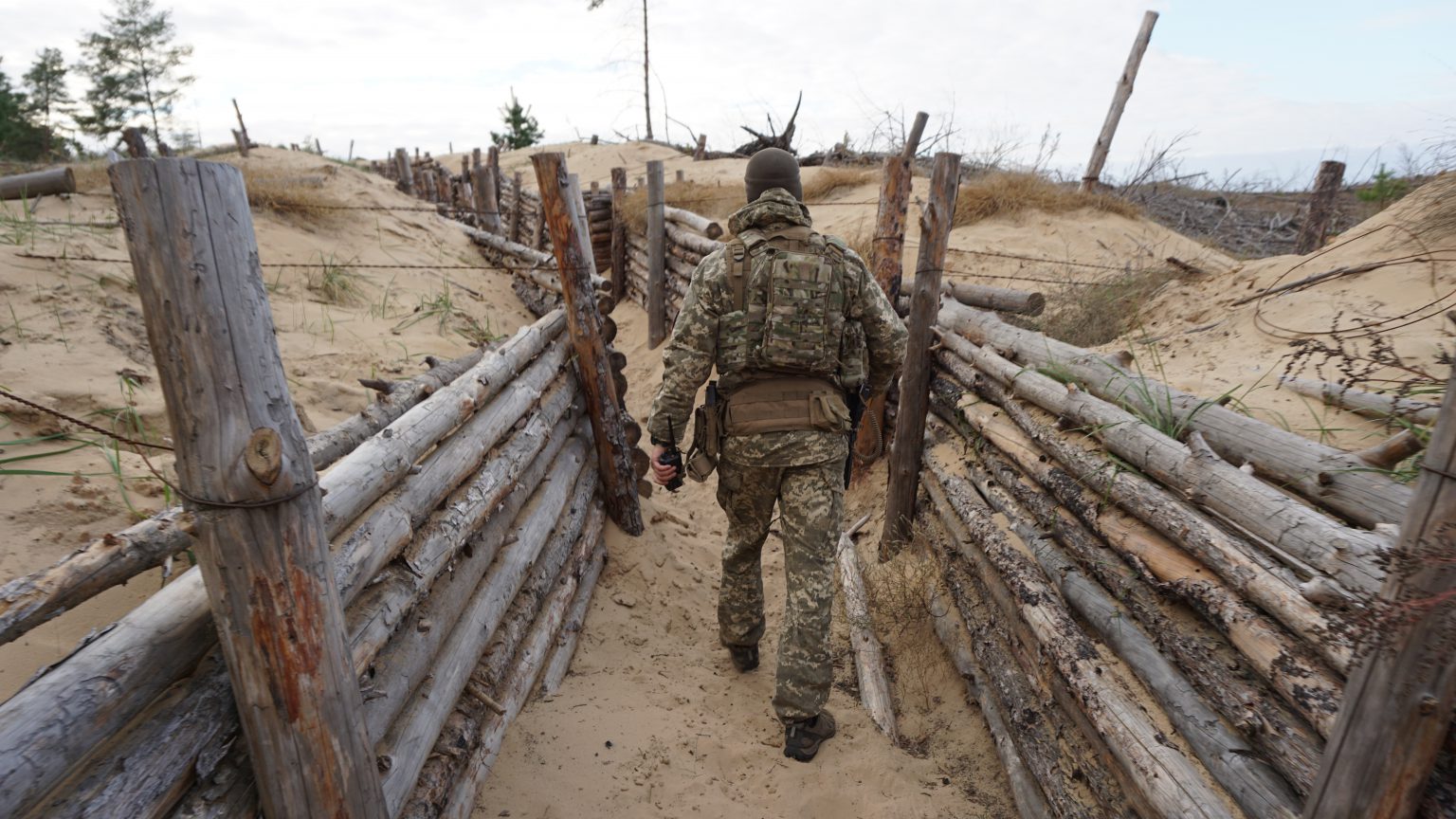In this wide-angle photo, a man named Holdger is walking through a military bunker alley or trench, characterized by sandy, tan soil. He is dressed in camouflage, possibly indicating he's a soldier or hunter, and wears a brown, thick belt around his waist. Visible from the back, Holdger also has boots and a knit cap. In his left hand, he is holding a walkie-talkie. The trench is constructed with parallel horizontal logs forming the walls, reinforced at intervals by vertical posts held up by wire cables to prevent caving. The walkway itself is made of sand or brown dirt, flanked by mounds of sand and sparse, leafless trees at a distance. Patches of brown grass dot the sandy hillsides, heightening the war-like, rugged ambiance of the scene.